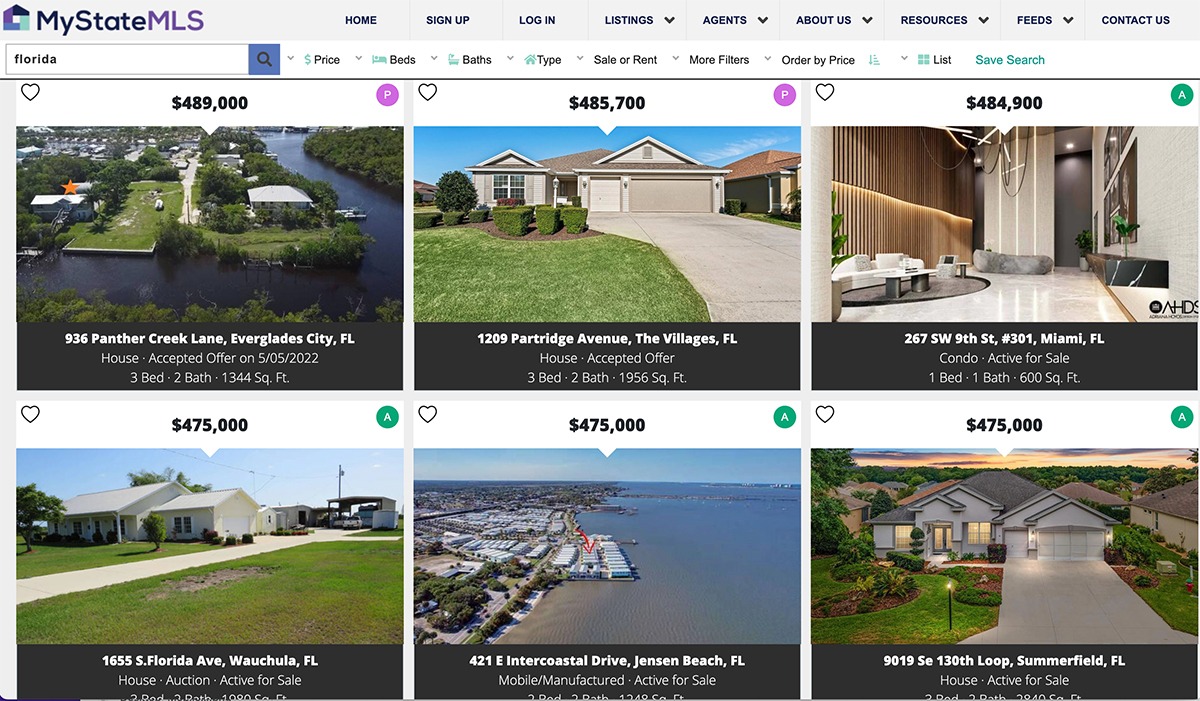The screenshot features the real estate website MyStateMLS, showcasing several property listings. One highlighted listing is a $489,000 house with a green exterior, situated beside a body of water. Another listing is a $485,000 large house with a tan driveway and a grassy yard. The $484,000 listing displays a luxurious kitchen. There is also a $475,000 sizable house with a green grass yard, a concrete driveway, and an exterior building. Additional $475,000 listings include a city port with part of the ocean and a large house with a well-maintained grassy yard and decorative yard lights. The website sports mostly black text, with a couple of pink or purple buttons at the top, set against a white background.